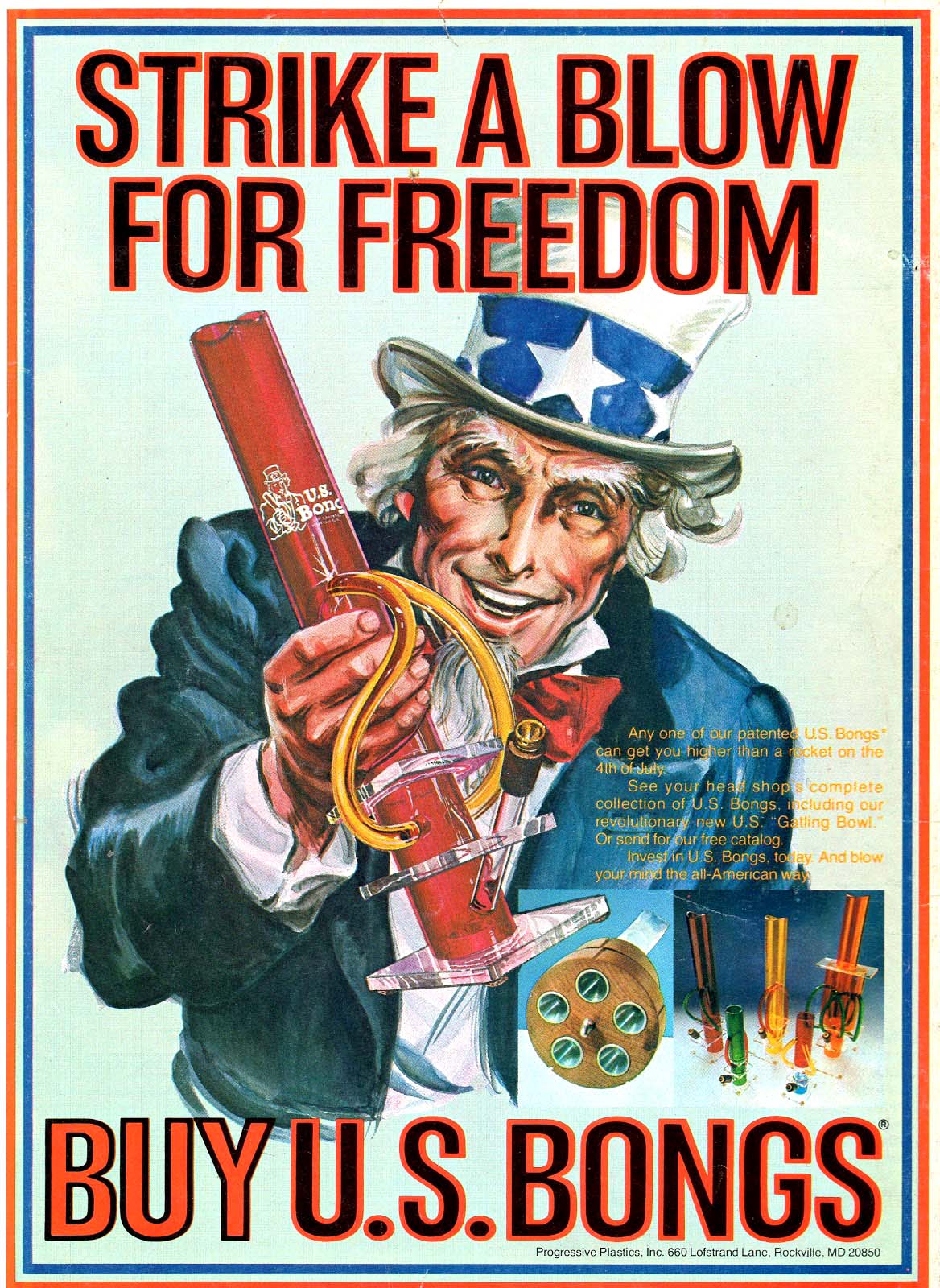This image is a vintage-style parody advertisement mimicking the classic Uncle Sam "I Want You" poster. In the center, a caricature of Uncle Sam, complete with his iconic white hair, bushy eyebrows, blue jacket, dress shirt, red bow tie, and patriotic hat adorned with stars, points directly at the viewer. His usual stern expression is replaced with a smile as he holds a red bong with yellow tubes and a white "U.S. Bongs" logo. Above him, the bold text reads "Strike a Blow for Freedom," and below, it says "Buy U.S. Bongs." To the side, an assortment of various bongs and accessories, including what appears to be a grinder, are neatly displayed in small boxes. A detailed, though small and hard-to-read, yellow text section boasts the product's efficacy: "Any one of our patented US bongs can get you higher than a rocket on the 4th of July. See your head shop's complete collection of US bongs, including our revolutionary US Gatling bowl or send for our free catalog. Invest in US bongs today and blow your mind the all-American way." The ad also includes the manufacturer's information: "Progressive Plastics, Inc., 660 Loft Strand Lane, Rockville, MD, 20850."